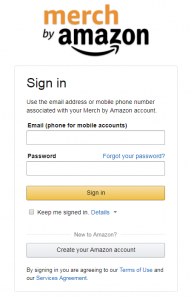The image appears to be a screenshot from a cell phone displaying the Amazon website, specifically the login page for "Match by Amazon". 

At the top of the page, the text "Match by Amazon" is prominently featured, with "Match" in orange and "by Amazon" in black, accompanied by Amazon's signature smiley face arrow logo. The entire layout is over a clean white background.

Below this header, there is a boxed section with the text "Sign in using the email address or mobile phone number associated with your Match by Amazon account", all in black ink. Following this, there's a text box labeled "Email (phone for mobile accounts)" where users can enter their credentials.

Further down, another text box labeled "Password" is provided, with the "Forgot your password?" link in blue ink adjacent to it. Below these fields, there's an orange button with the label "Sign-In" in black ink.

Additionally, there is a "Keep me signed in" checkbox option, accompanied by a "Details" link in blue ink. 

For new users, the page offers a "Not new to Amazon? Create a new Amazon account" option. At the bottom, there's a disclaimer stating, "By signing in, you agree to our Terms of Use and our Services Agreement."

Overall, the image depicts a straightforward and user-friendly interface designed for easy login and account management on Amazon.